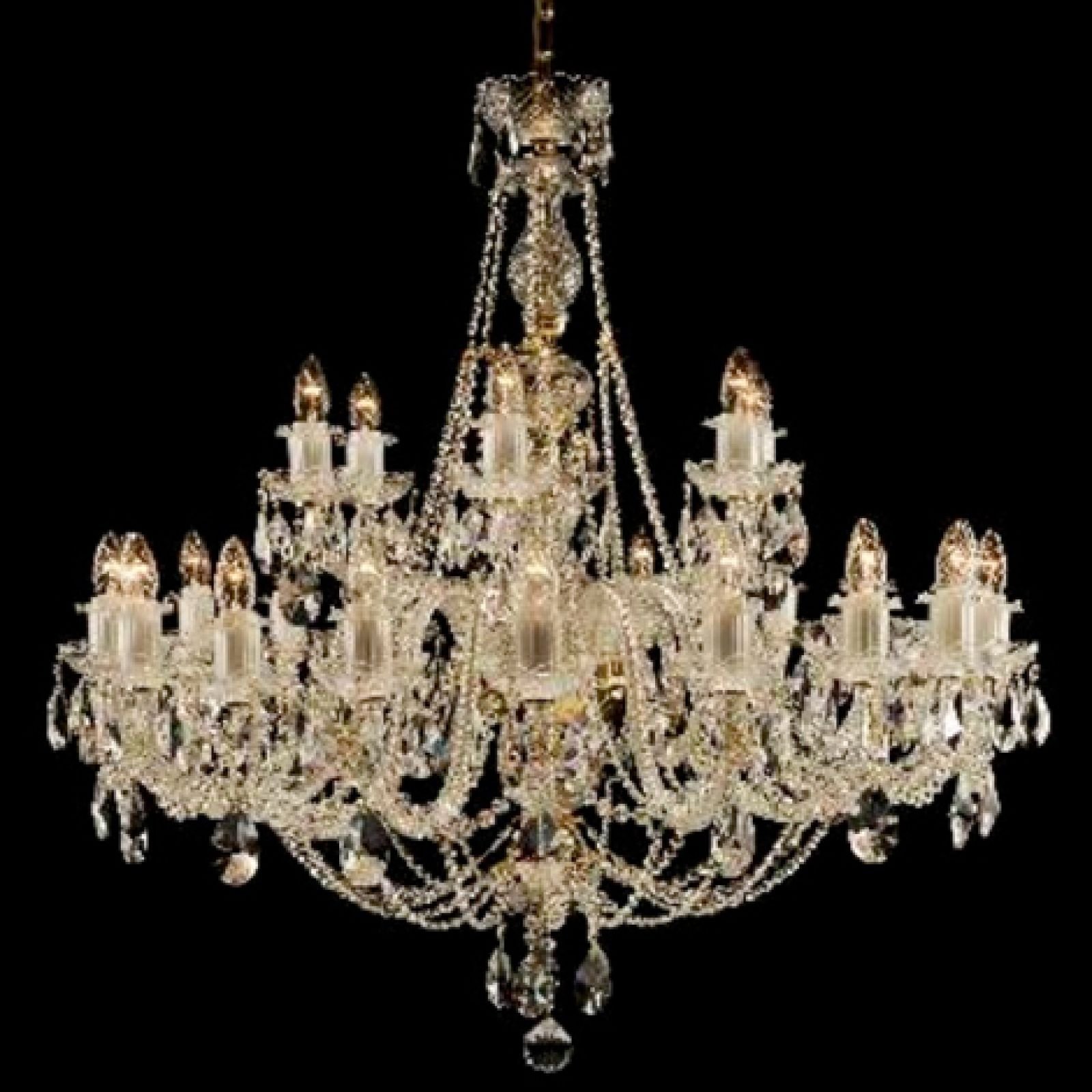This close-up digital photograph captures an ornate and delicate glass chandelier set against a completely black background. The chandelier features two tiers of candle-shaped lights, with a larger ring of lights on the lower tier and a smaller ring on the upper tier. Each light resembles a glass candle with a candlestick and is supported by a little glass saucer. Interconnected by strands of round, pearl-like clear balls, the lights emit a soft yellow hue. Dangling teardrop crystals and chains of crystal adorn the chandelier, which is held up by a brass-colored metal rod and chain. The intricate detailing includes multiple layers of finely crafted glass beads and other delicate decorations, creating a stunning visual display.